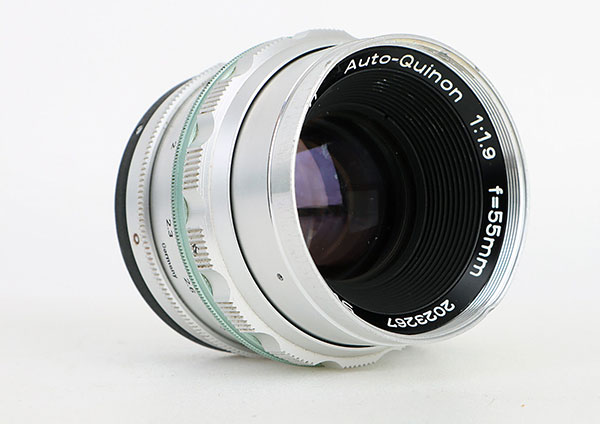The close-up image depicts a professional telephoto camera lens positioned against a white rectangular background, likely a light box. The lens is primarily metallic silver with various intricate features including several textured rings, some of which have raised rectangular platforms for adjusting focus and zoom. There is a black ring at the base where the lens would connect to the camera, and a light green or mint blue ring encircling the middle. The lens's outer structure consists of multiple numeric markings such as 2, 2.3, 2.6, often used for precise adjustments. The interior of the lens reveals ridged black details extending almost to the outer edge, with the reflective glass lens prominently visible in the center. On the front border of the black circle, in white lettering, it reads "Auto Kinyon 1:1.9 F=55mm," along with other numeric inscriptions like 2.0, 2.3, 2.6, 7, detailing aperture and measurement specifications.